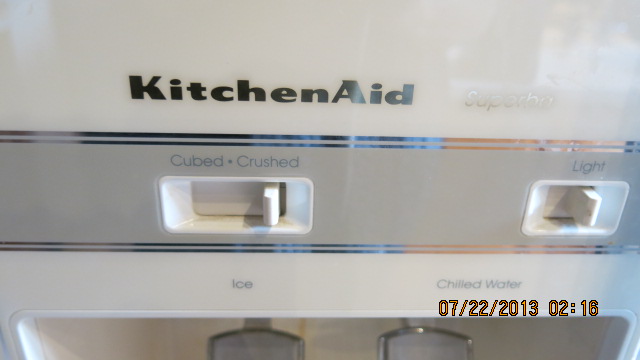This photograph captures a KitchenAid appliance, likely an automated ice maker or refrigerator, prominently displaying the KitchenAid logo at the top. The appliance is beige with a distinctive black stripe running through the middle. On the right, an additional label, possibly reading "Superba," is visible. The main control panel features options for either cubed or crushed ice next to a slide button. Currently, the setting is adjusted to "crushed." Further right, there's a light button, which is switched to "on." Below these controls, there are clearly marked areas for dispensing ice and chilled water. The dispensing mechanism includes a metal lever or pedal that is pressed by a cup to dispense the selected option. The controls and buttons have a gray stripe with two silver pinstripes behind them. Additionally, the photograph bears a timestamp in orange, reading "7-22-2013 at 2:16 a.m."